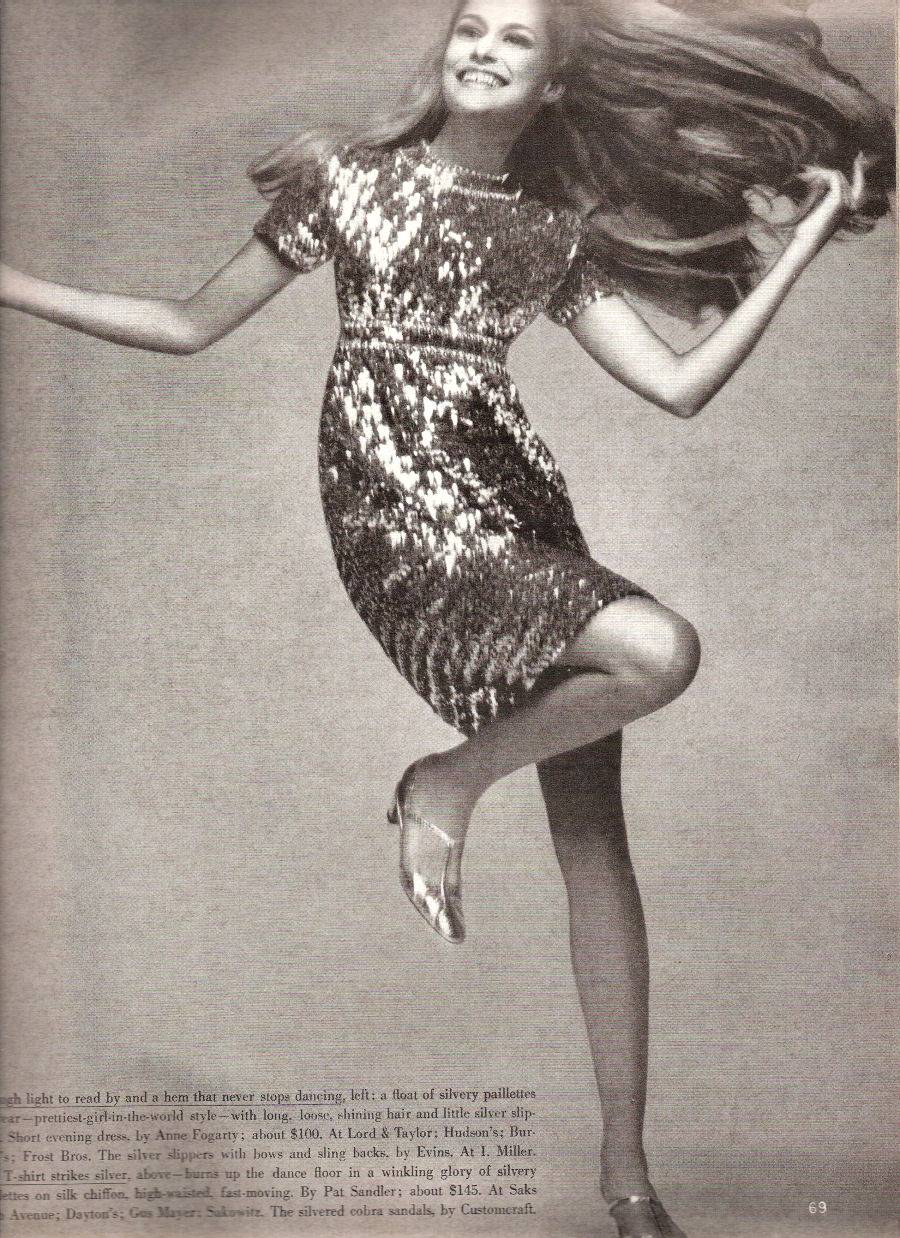This black and white photo, likely from a magazine, captures a young Caucasian woman mid-dance, radiating joy with a beaming smile. She wears a knee-length, short-sleeved dress entirely adorned in sequins, with a distinctive pattern of sequins or rhinestones accentuating the empire waistline and neckline. Her long, flowing hair is caught in motion, as her left hand playfully lifts it, and her right leg is bent and lifted, suggesting movement. She completes her sparkling ensemble with shiny silver heels. The image, potentially an advertisement or a celebrity feature, includes a partially obscured caption in the lower left corner detailing elements of her wardrobe, such as the short evening dress designed by Ann Fogarty priced around $100 at Lord and Taylor. Page number 69 is visible near her foot, indicating its placement within the magazine.